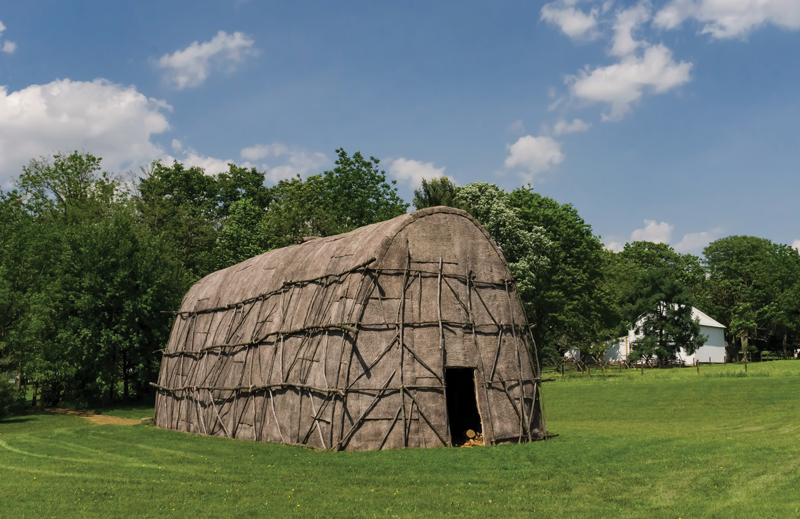The image depicts a large, cylindrical hut-like structure with a rounded roof, situated in a well-kept grassy field. The hut, estimated to be about 16 feet tall and 35-40 feet wide, is constructed from a brown or gray canvas fabric, supported externally by wooden sticks or poles, giving it a rustic, organic appearance. The front of the hut features an open doorway with no apparent means of closure. To the right of the structure, partially obscured by approximately seven trees, is a white house, seemingly separated from the hut by a fence. Additionally, there appears to be a log or piece of wood near the entrance of the hut. The scene is set under a partly cloudy, blue sky, indicating a sunny summer day.